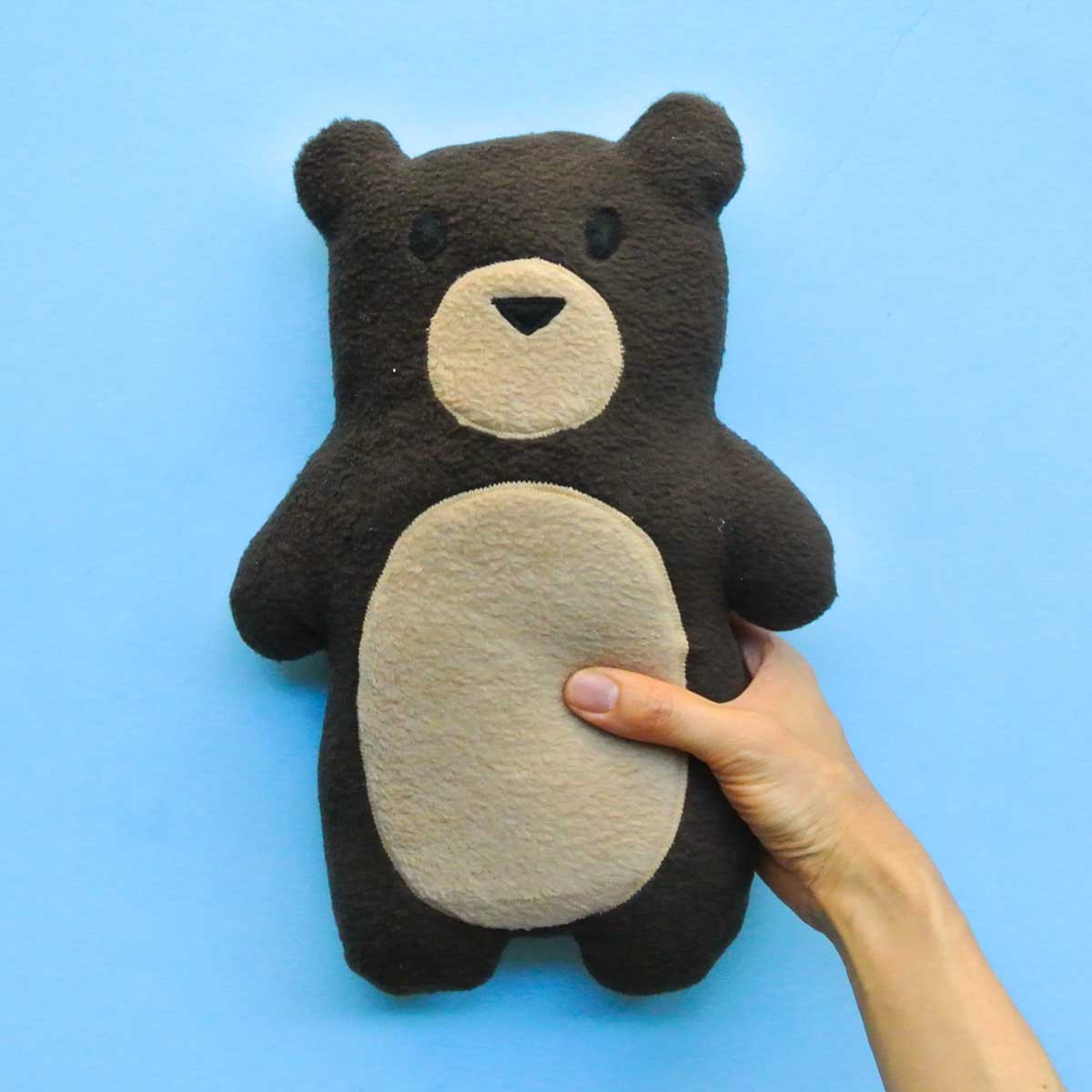In the image, a dark brown to almost black, homemade stuffed teddy bear is held against a light powdered blue background. Unlike traditional teddy bears, this one is flat like a pillow. The bear has a distinctive design with a felt tan panel on its belly and a matching tan muzzle. Its facial features include two dark black button eyes and a black, upside-down triangular nose. The bear's mouth area is signified by a large circular tan felt area surrounding the nose. A person's lower arm and hand, appearing Caucasian, extends from the bottom right of the image, holding the bear in place. The hand wraps around the bear, with the fingers positioned behind the bear's hip area and the thumb lying across its belly, almost touching the center of the tan felt panel. The visual simplicity and homemade charm of the bear stand out against the vibrant blue background, highlighted by the contrasting colors and textures.